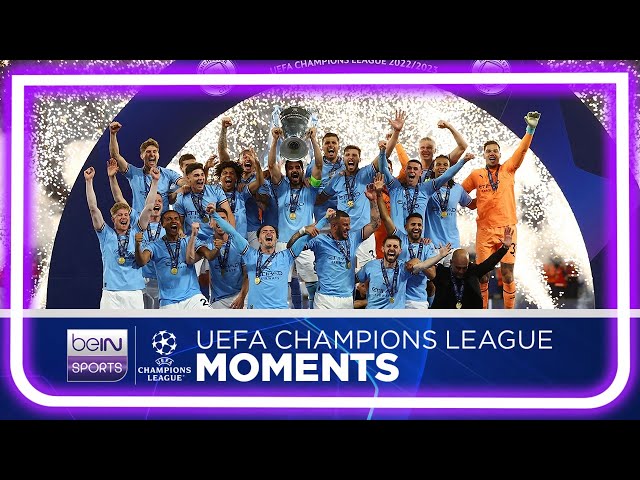The photograph features a triumphant sports team celebrating a UEFA Champions League victory against a black background. Encased by a glowing white and purple neon border, the image captures the jubilant moment. At the center, a player hoists a large silver trophy high in the air, surrounded by teammates all wearing light blue jerseys and gold medals on blue ribbons. Their arms are raised in celebration, and fireworks illuminate the background. A few players on the right side are dressed in all orange, while a man in a black suit stands in front with his hands up. The bottom of the image displays text: "Be In Sports, Champions League, UEFA Champions League Moments," accompanied by the Champions League star logo.